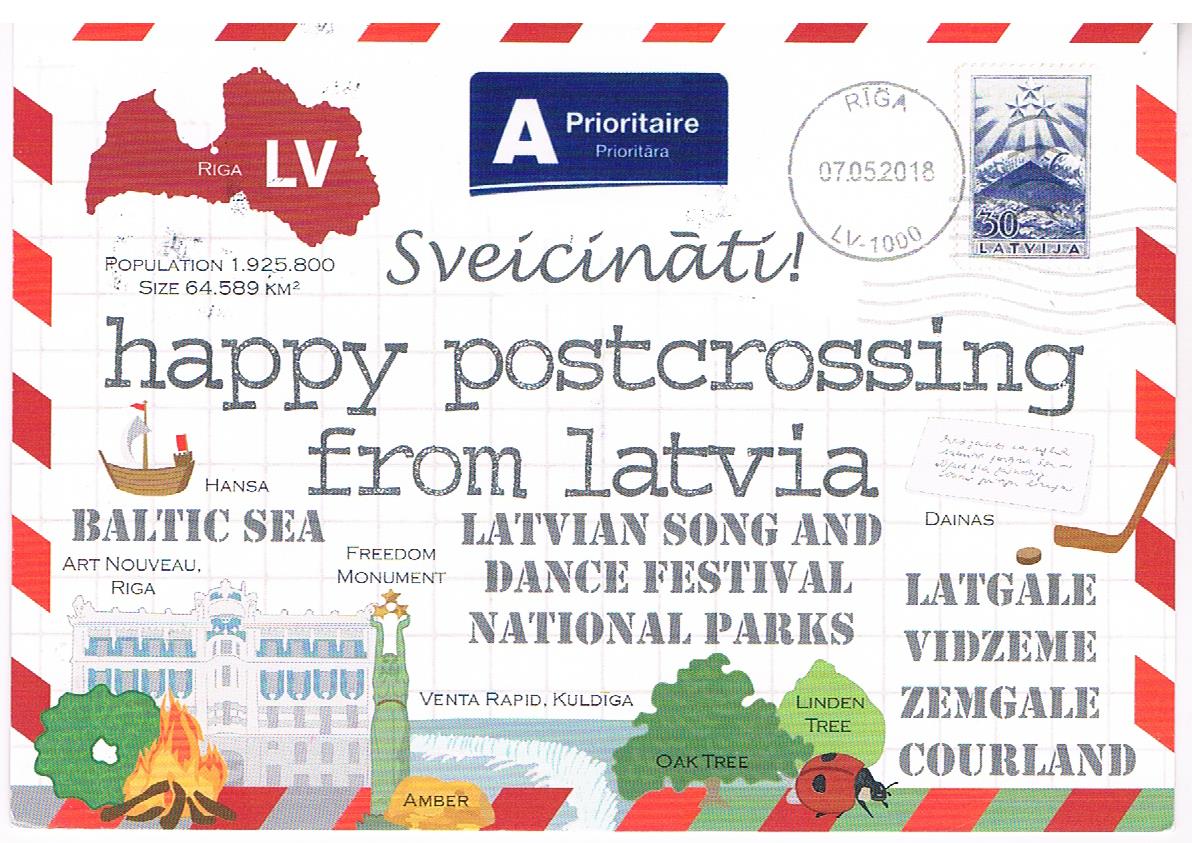This detailed promotional postcard from Latvia, designed to resemble an old-fashioned airmail envelope, features a striking red and white striped border. Centrally, it proudly carries the greeting "Happy Post Crossing from Latvia," followed by a depiction of the Latvian population and size statistics. A prominent "Riga LV" logo occupies the top left, while the top center boasts the word "Prioritaire" in a blue rectangle. The upper right corner showcases a postmark dated 07-05-2018 from Riga, LV1000, alongside a blue and gray postage stamp.

The postcard weaves cultural and natural imagery throughout. The bottom left corner portrays a campfire graphic beside the word "Baltic Sea" and a small image of a boat labeled "Hansa." Above "From Latvia," there's a symbolic illustration of the Freedom Monument, indicating the rich heritage of Latvian Song and Dance. The handwritten-style script "Sveicināti!" adds a warm touch.

Complementing these visuals, the lower part of the postcard lists various regional names: Latgale, Vidzeme, Zemgale, and Courland. Surrounding these are illustrations of indigenous trees like oak and linden, along with a ladybug, emphasizing Latvia's natural beauty and biodiversity. This multifaceted, illustrated postcard captures the essence and cultural richness of Latvia.